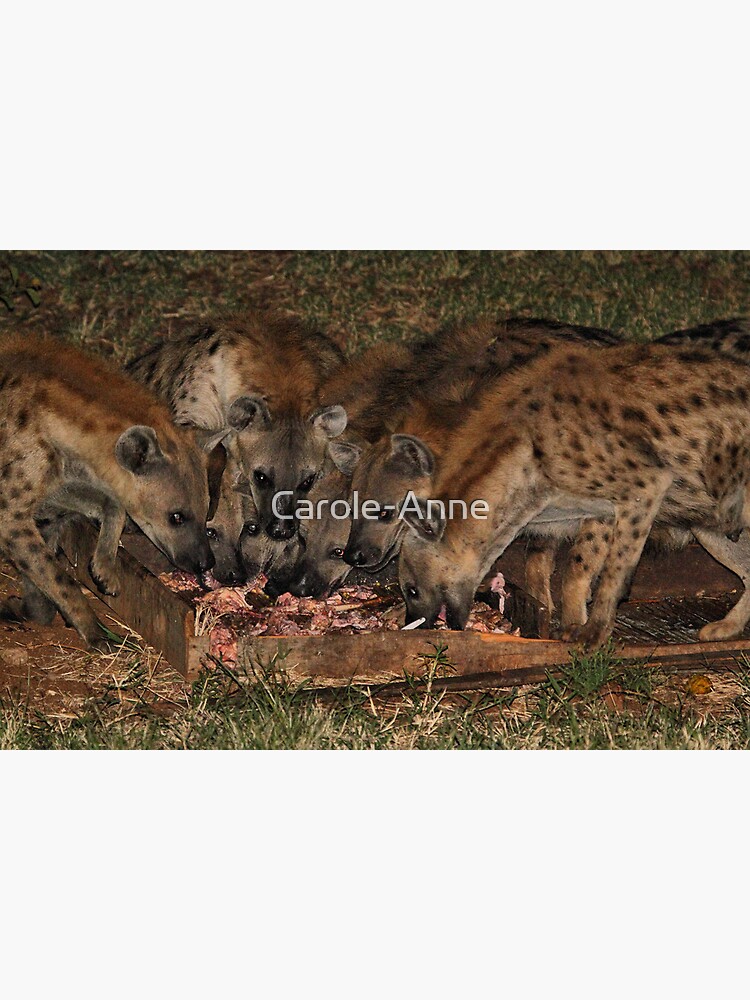A detailed drawing depicts a cluster of at least seven hyenas devouring an animal carcass from a flat wooden trough in a grassy area. These hyenas, characterized by their distinctive dark brown necks, lighter bodies with black spots, and two-tone faces featuring darker hues around the eyes and noses, are all hunched over their meal. One hyena on the left looks rightward, while others are positioned forward and coming in from the right. The scene teems with raw energy as the hyenas tear into the meat and bones, framed by the grassy ground beneath them. The image also features a watermark at its center reading "Carole-Anne," indicating the artist or photographer's name.